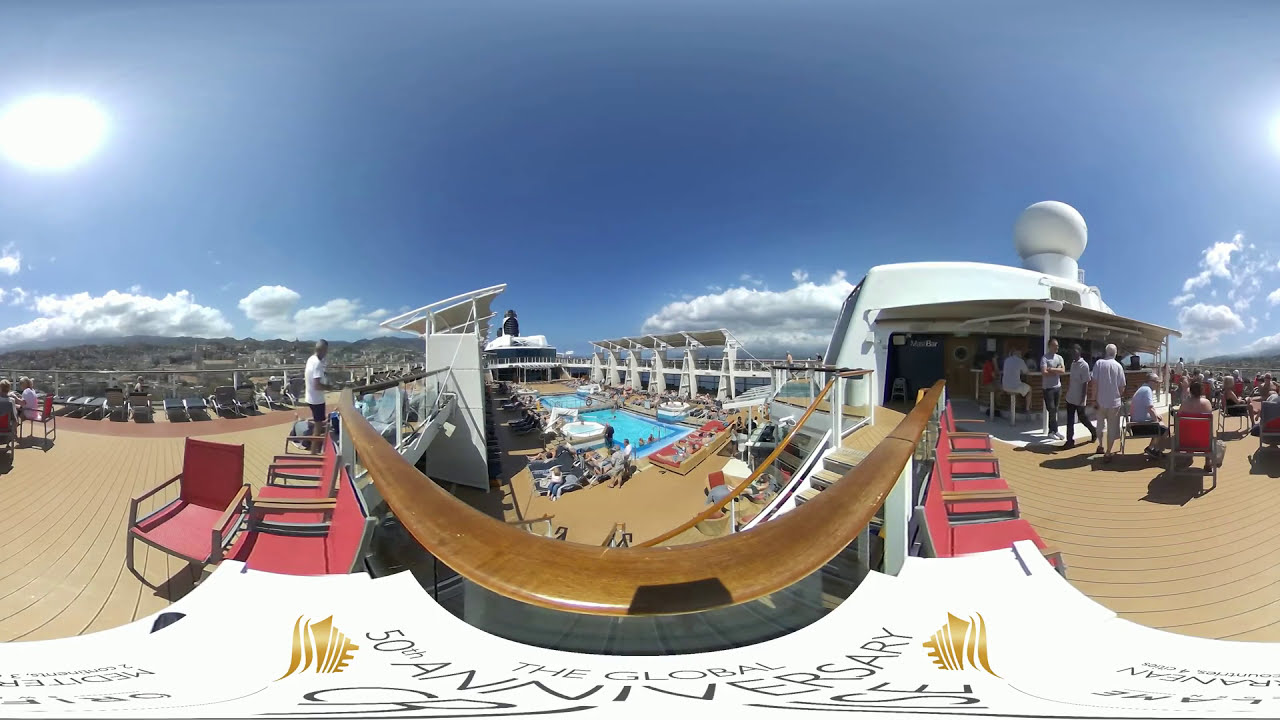The image captures the vibrant, sunlit top deck of a cruise ship celebrating "The Global 50th Anniversary Cruise, Mediterranean." At the front of the picture, partial signage indicates this special occasion. The deck features an array of red beach chairs with wooden handles, which are occupied by numerous sunbathers. Some people are seen standing by the railings on both the left and right sides of the ship, while others are seated or mingling by a bar on the right. Below, on the deck centered under the top deck, lie two swimming pools surrounded by additional beach chairs and numerous people lounging and swimming. The flooring appears to be wooden, while the ship itself is white. The backdrop reveals distant mountains under a bright blue sky punctuated by a few white clouds and a radiant sun.